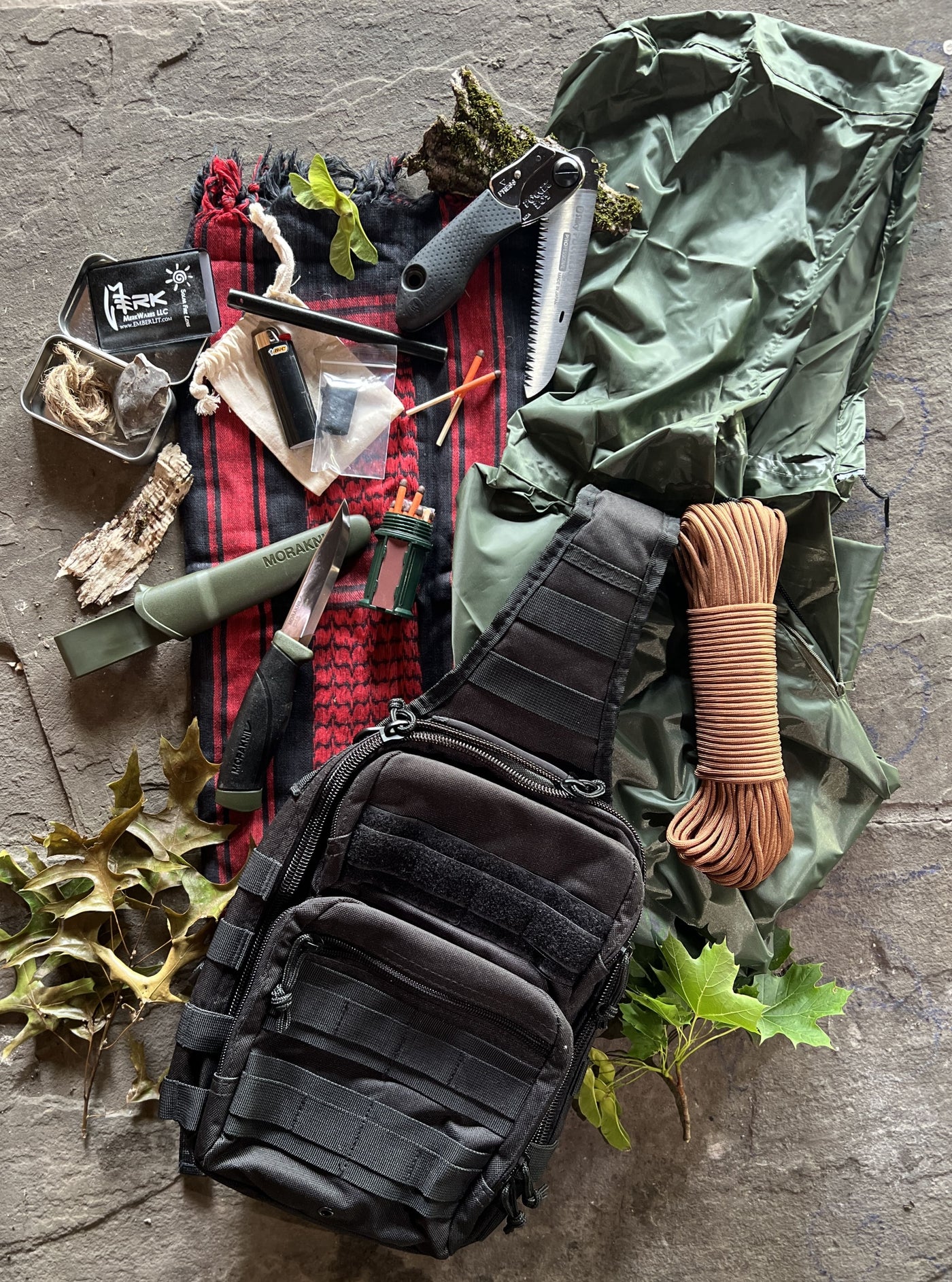The vertical rectangular photograph captures an overhead view of a green duffel bag, open and spilling its contents across a gray flat stone surface, suggesting an outdoor setting. The bag features an open side zipper and a red plaid interior lining, with a separate compartment at the top housing various smaller pieces of equipment. Spread around the bag are various camping tools: a brown coiled rope peeking from an additional top pocket, a foldable saw, a sharp knife with a black handle, and a green-handled tool. An open black container lies nearby, holding extra string and other miscellaneous items. Also notable are a black over-the-shoulder backpack and a small black lighter positioned on a red and black fringed blanket that partially covers the stone surface. Scattered around are leaves and seeds, adding a natural touch to the scene.